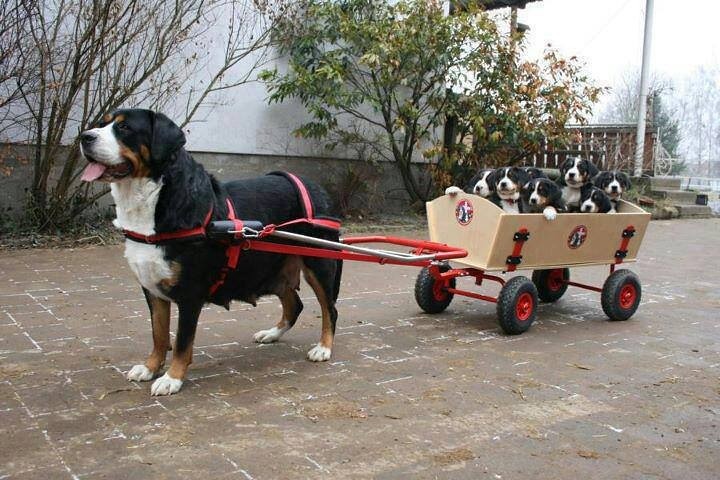This photograph captures a large St. Bernice mountain dog with a black back, white paws, and black and brown legs. Her coat features a white throat and chest, black ears, and fur around her eyes, along with a white muzzle accented by brown markings on the sides of her face and a dark nose. The dog, with full teats visible, stands on all four legs on a paved or cobblestone courtyard with her mouth slightly open and tongue hanging out, seeming to smile. She is connected to a blonde wood cart with red hardware and four black and red rubber tires via a red harness system. The cart is laden with approximately seven puppies, presumably her own, sharing her black, white, and brown coloring. The puppies, appearing of the same breed, stand with their little paws hanging over the edge of the cart, eagerly looking out. The scene unfolds next to a white house with a small porch and a few sparse trees in the background.